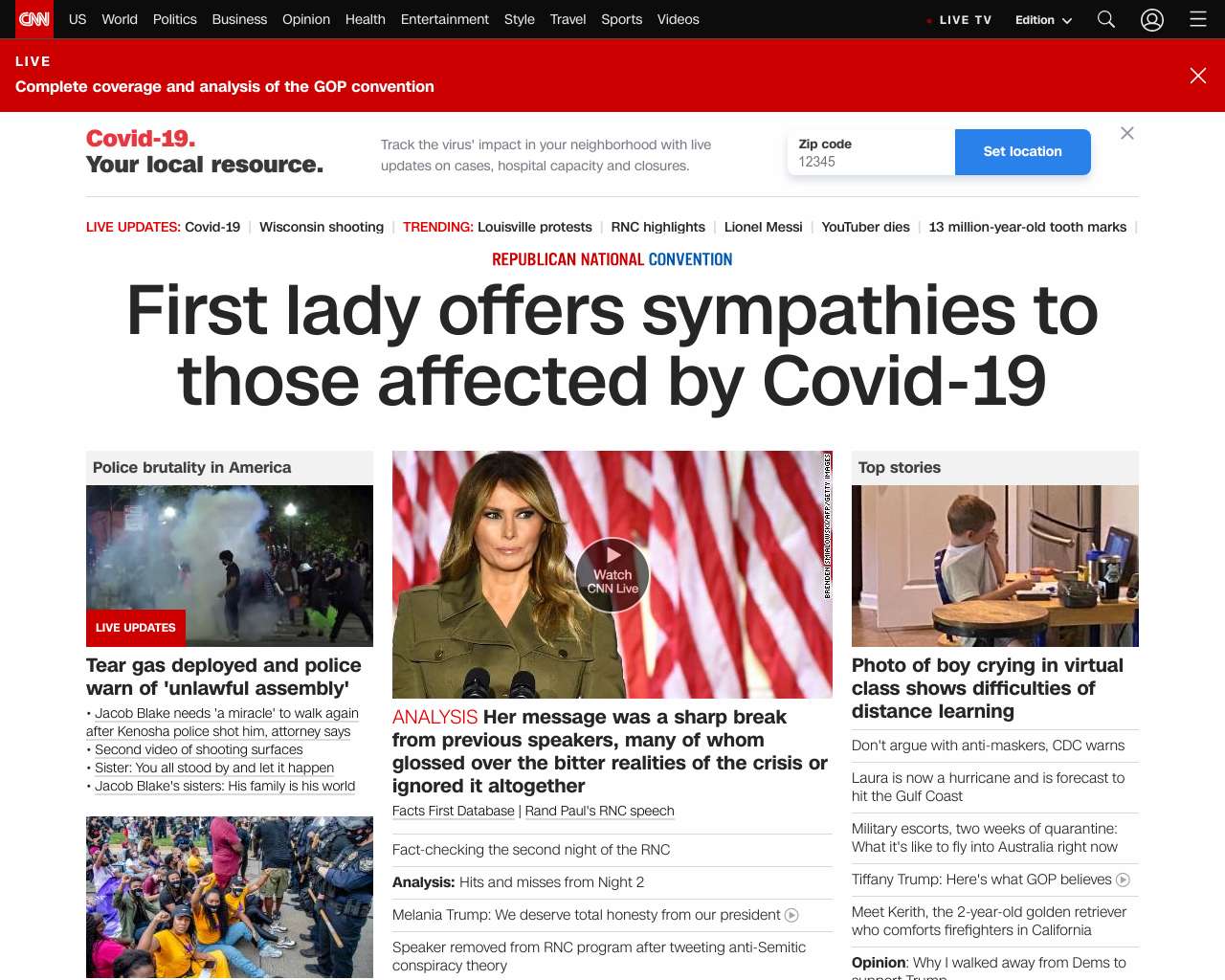The image is a detailed screenshot of the CNN homepage, specifically focusing on news related to U.S. politics. At the top, a black banner spans across the screen, prominently displaying the CNN logo on the left in its iconic red and white. Adjacent to the logo are navigation links including U.S., World, Politics, Business, Opinion, Health, Entertainment, Style, Travel, Sports, Videos, and Live TV Edition, accompanied by a user account icon and a search icon shaped like an hourglass. The "CNN" link is highlighted in red, indicating the current section.

Immediately below, a red bar announces "Live Complete Coverage and Analysis of the GOP Convention," signifying that the page is focused on political coverage. Visible article headings predominantly mention the Republican National Convention, with key words "Republican" and "National" highlighted in red, while "Convention" stands out in blue.

The main headline, written in large, bold text, reads "First Lady Offers Sympathies to Those Affected by COVID-19." To the left of this headline, there is an image of a man enveloped in what appears to be tear gas, labeled with "Live Updates" and captioned "Tear Gas Deployed and Police Warn of Unlawful Assembly." 

In the center of the page, there is a picture of the former First Lady, Melania Trump, labeled with "Analysis" in red. The accompanying text notes that her message represents a significant departure from previous speakers, who either glossed over or ignored the harsh realities of the COVID-19 crisis.

On the right side, an image depicts a young boy sitting at a desk, seemingly distressed with his face buried in his short-sleeved white shirt. The caption for this image reads "Photo of Boy Crying in Virtual Class Shows Difficulties of Distance Learning." Next to the boy is a smaller wooden stool.

Additionally, there is a circular icon reading "Watch CNN Live," indicating the presence of a live video stream. The rest of the text is too small to decipher, but the overall layout and headings confirm the page as an online news site, specifically CNN, offering comprehensive news coverage.